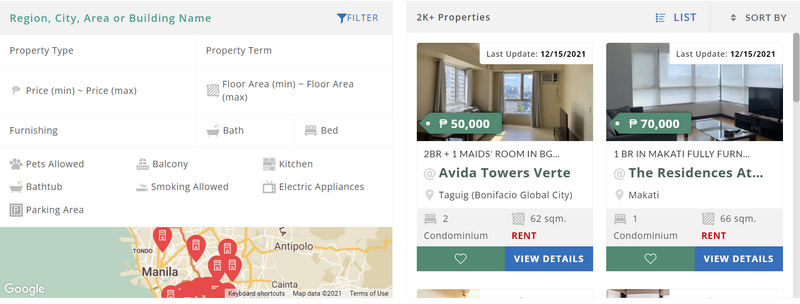This is a detailed screenshot of an apartment rental app or website. In the upper left corner, it displays the region, city, area, or building name. A prominent blue-colored button labeled "Filter" is situated towards the middle of the screen. In green letters, the initial region, city, area, or building name is highlighted, while in black letters, the text "2000 UK, UK plus properties" stands out. On the upper right corner, there's a blue "List" button and a "Sort by" dropdown menu in black letters. 

Along the left side of the page, several filtering options are presented: "Property Type" and "Property Term" are at the top, followed by "Pricing Minimum" and "Maximum," and "Floor Area Minimum" and "Maximum." Below these, additional parameters include "Furnishing," "Bathrooms and Bedrooms," "Pets Allowed," "Bathtub," "Parking Area," "Balcony," "Smoking Allowed," "Kitchen," and "Electrical Appliances." 

Below the filtering options, there's a map showing the selected city, which appears to be Manila. On the right side of the page, two property listings are visible: "La Vida Towers Verde" and "The Residence at..."